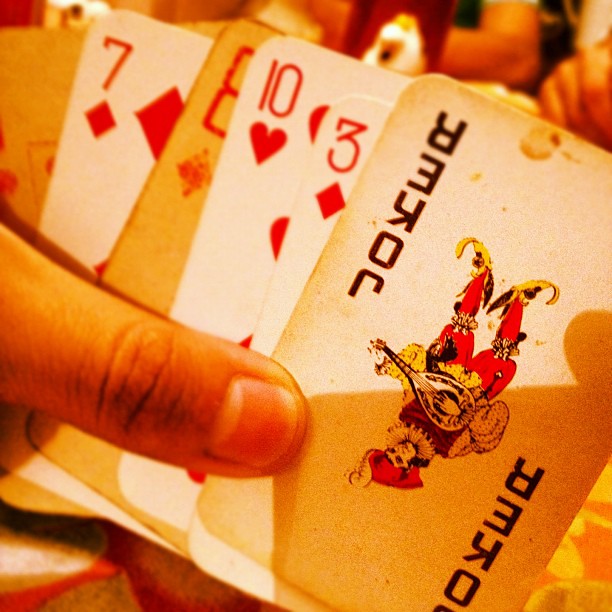This vivid close-up photograph showcases a hand delicately gripping a fan of playing cards. The visible cards include the 7 of diamonds, 8 of diamonds, 10 of hearts, 3 of diamonds, and a distinctive joker. The joker card, notable for its inverted orientation, depicts a skeletal figure holding a lute, adding a quirky, eerie touch to the image. A shadow casts across the bottom right quadrant of the joker card, enhancing the photograph's depth. The backdrop, rendered in warm, orange, and red tones, features blurred silhouettes of people, creating a lively yet indistinct setting. To the right of the joker card, a hint of an orange and white surface peeks through, offering a glimpse into the scene's broader context. The overall ambiance of the photograph is naturally suffused with an orange-yellow hue, lending a nostalgic, almost sepia-like quality to the composition.